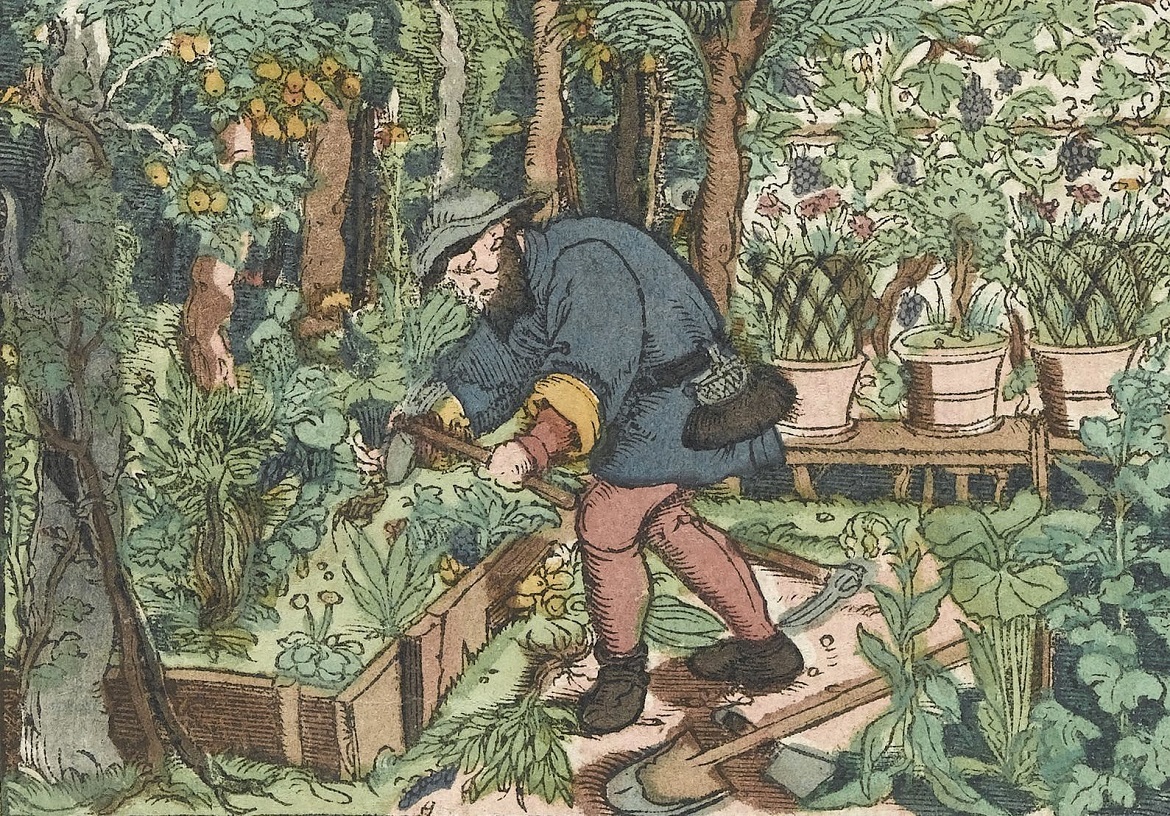This illustration, likely a watercolor painting, vividly captures a bearded man immersed in gardening within a lush, garden-type landscape. The man, distinguished by his wide, double-pointed beard and gray hat, wears a loose-fitting blue tunic with rolled-up sleeves, brown pants, and dark brown boots. A belt with a bag is fastened around his waist. He is hunched over a wooden raised garden enclosure, approximately 12 to 15 inches high, which contains green leafy vegetables and cabbages. In his left hand, he holds a gardening tool, possibly a hoe, as he appears to be harvesting or tending to the plants within the enclosure. 

At his feet lies a shovel and a pick. Behind him, there are numerous additional pots with small trees and plants, including a lemon tree bearing fruit and other various trees that may have oranges. The background features a dense array of green plants and another darker patch of ground with more green leafy vegetables, enhancing the scene's rich, botanical ambiance.